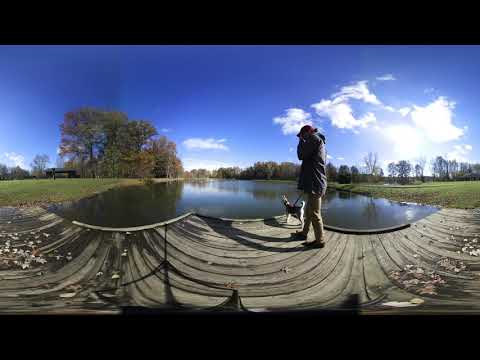This panoramic photograph, captured with a fisheye lens and distorted for a 360-degree view, features a man standing on a wooden dock or bridge extending over a small, reflective body of water, possibly a pond or a narrow river. The man, wearing a blue top, beige pants, and a hat, is holding a small brown and white dog on a leash. They both look out over the serene, still water, which mirrors the blue sky and white clouds above. A green field with scattered leaves borders the dock, with tall trees to the left and a mix of smaller, barer trees and bright sunshine on the right. There is a man-made structure partially visible on the left, though its purpose is unclear. The scene is framed by black bars at the top and bottom, suggesting the image is a still from a video, and the curvature of the image heightens the immersive, expansive outdoor setting.